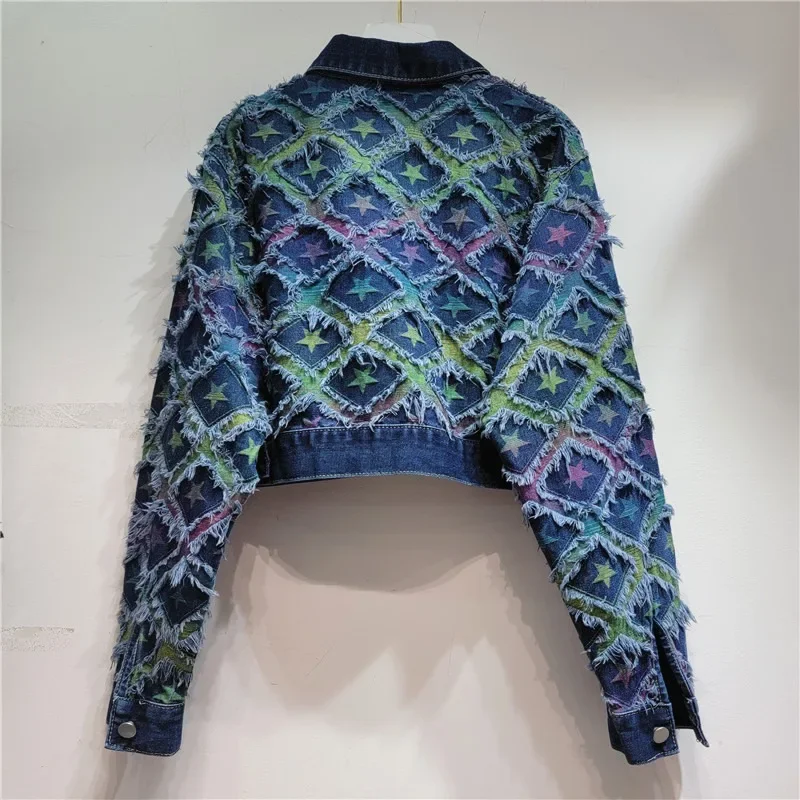The image shows a highly detailed, intricate denim jacket hanging on a white or very light-gray wall, emphasizing a sense of minimalistic backdrop to highlight the garment. The jacket, displayed almost as if it were an art piece, is suspended by a gold hanger. The overall view is from the back, showcasing the elaborate design. The denim is dark blue, forming a collar, waistband, and cuffs. The main body of the jacket features a grid-like pattern of diamond-shaped panels with frayed edges. Each panel is filled with colorful stars in light green, pink, dark blue, and purple, creating a vibrant and whimsical mosaic. The sleeves, extending long and adorned with the same star-studded diamond patterns, amplify the jacket's fanciful design. Shadows from the jacket cast subtle details on the wall, enhancing the textural depth of the image.